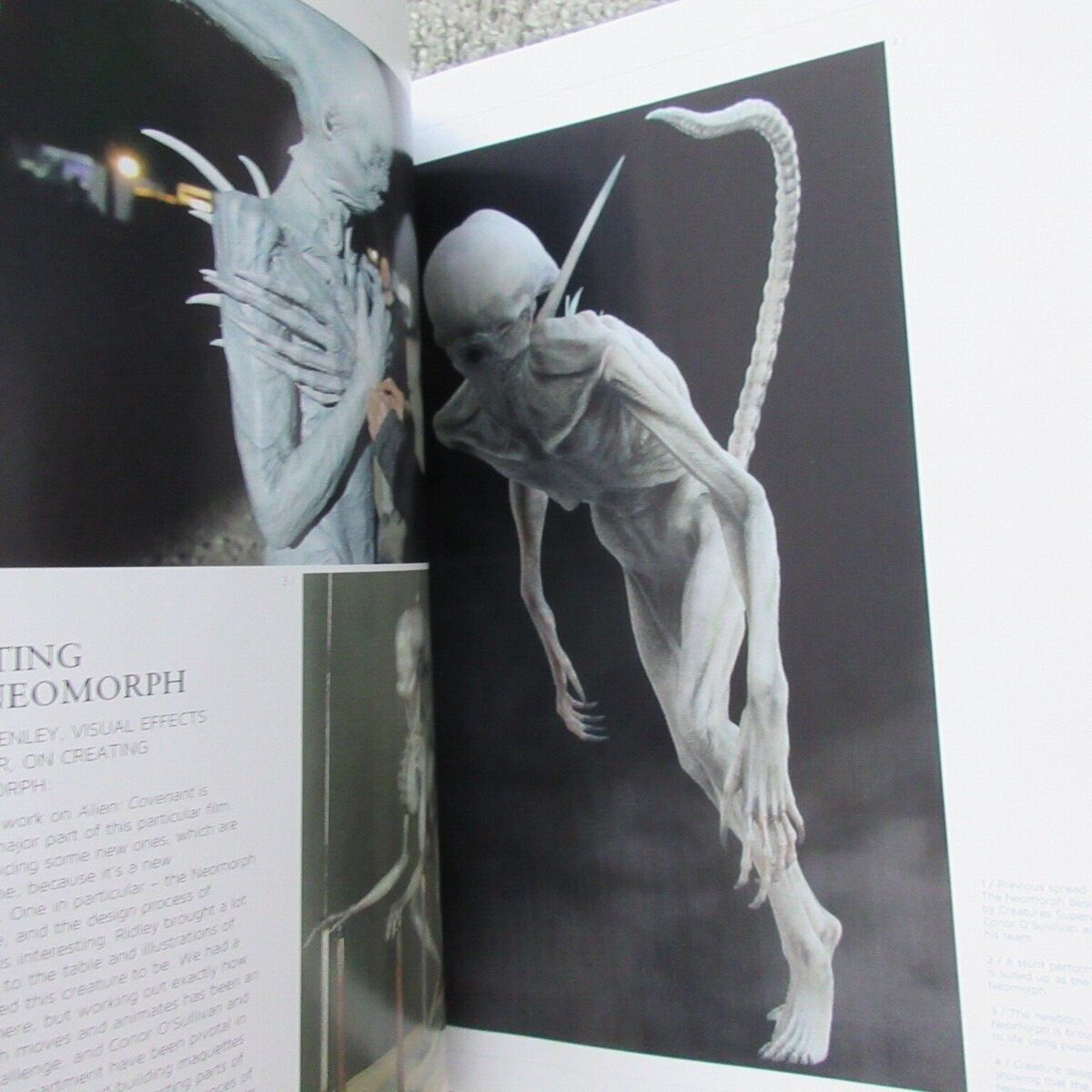In this photograph, we see an open book displaying two pages filled with detailed illustrations and text. The right-hand page is dominated by a full-page drawing of a fantastical alien creature. This creature has an eerie, almost human-like form, with long gangly arms, sharp nails, and a lengthy tail that arcs gracefully from its back. Strikingly light gray in color, the alien stands out against the dark black background. Its head is elongated, without visible eyes but featuring a menacing mouth. The alien’s feet are somewhat humanoid, adding to its unsettling appearance.

The left-hand page offers a mix of text and illustrations. At the top, there is a smaller picture of another monstrous figure, also white and fantastical, displaying long fangs and crossed hands. Additional images accompany an article on the left side of this page. While predominantly black and white, the left page features hints of color interspersed within the text and illustrations. The page appears slightly bent back, making the right page more prominently visible. This book or magazine appears to be dedicated to the depiction and description of these imaginative alien creatures.